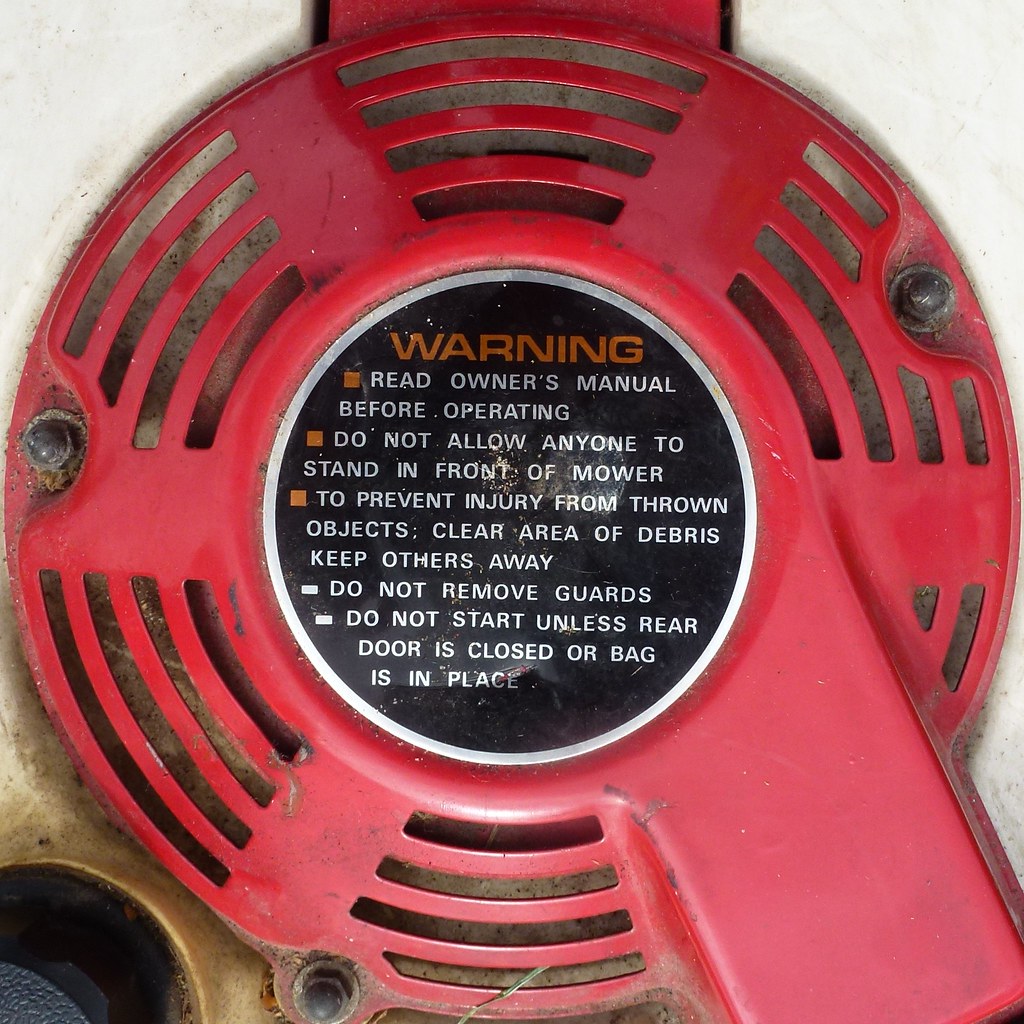The image depicts a close-up of the warning label on a red, metallic, fan-shaped component of a lawn mower. The component has vents and spaces within the red metal parts. Dominating the center is an oval-shaped, black circle with a silver border. At the top of this black circle, the word "WARNING" is prominently displayed in orange letters. The label contains detailed safety instructions in white text, advising users to read the owner's manual before operating, to keep others away and clear the area of debris to prevent injury from thrown objects, to not remove guards, and to ensure the rear door is closed or the bag is in place before starting the mower.